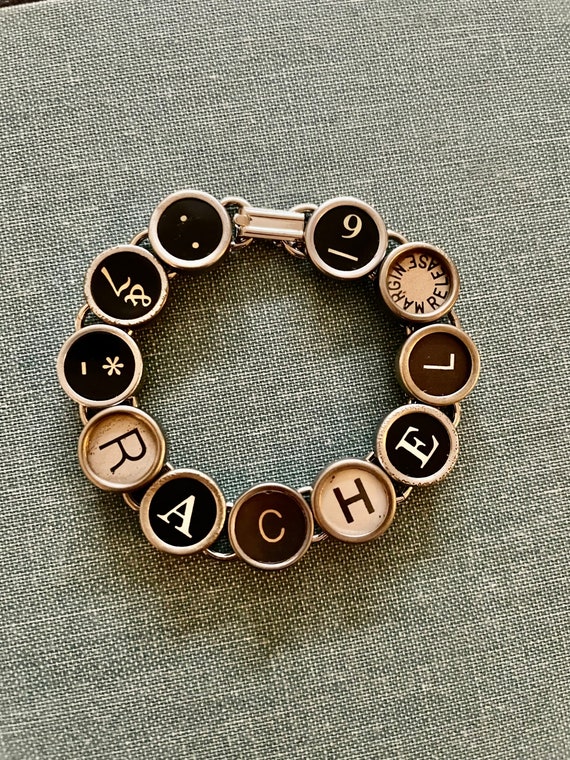The photograph features a distinctive bracelet composed of old typewriter keys, arranged to spell out the name "Rachel" (R-A-C-H-E-L). Each typewriter button, encased in a silver rim, showcases a different font and background color, ranging from black and white to dark brown. To fill out the bracelet, additional keys displaying various symbols—such as an asterisk, a colon, a seven, and a nine—are interspersed among the letters. The bracelet is designed with a silver clasp and is neatly arranged on a piece of gray fabric. This unique piece of jewelry combines nostalgia and personalization with its eclectic mix of typewriter keys and symbols, harmoniously set against a monochromatic backdrop.